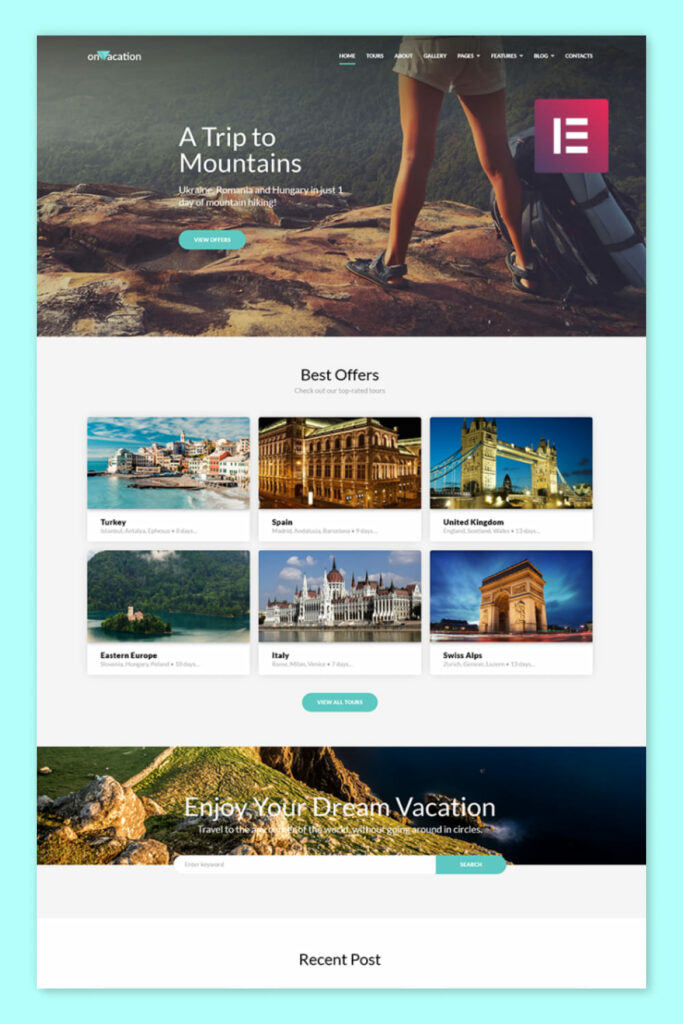Screenshot of a mobile-optimized webpage with a light teal background. At the top of the screen, an image shows a person standing on the edge of cliffs overlooking the water, with a backpack placed by their legs. Text overlays on this image read "A Trip to the Mountains" and a teal button beneath it that says "View Offers." In the same image box, "On Vacation" is displayed in the upper left corner. 

To the middle right, there are clickable word options, and "Home" is currently selected. Beside the "Home" tab, seven additional navigational tabs are visible.

Next to the person's backpack, there is a burgundy square with a white letter 'E' inside it. Below this section, there are highlighted "Best Offers" presented in two rows of three pictures each, showcasing various travel destinations:

Top Row:
1. Turkey
2. Spain
3. United Kingdom

Bottom Row:
1. Eastern Europe
2. Italy
3. Swiss Alps

At the bottom of the screenshot, a banner displays an image captioned "Enjoy Your Dream Vacation."